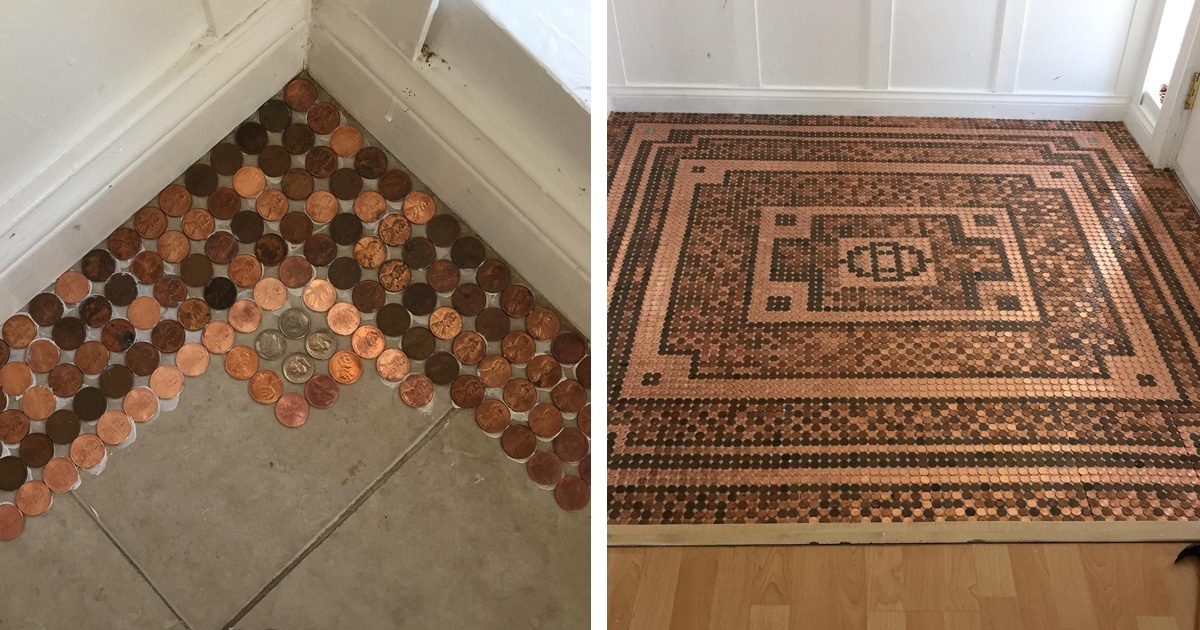The two square images together form a landscape layout, capturing the intricate process and the final artwork of a penny rug tile design. The left image zooms in on a corner of a room, showcasing a cream-colored tiled floor with brownish-grey grout and a white skirting board against white walls. Various shades of pennies, ranging from bright and shiny to dark, have been meticulously glued down in neat rows along the wall. A small square arrangement in the corner features four quarters, highlighting the detailed layout in progress, with visible white adhesive surrounding the coins.

The right image provides a zoomed-out view, revealing the completed mosaic. The design, set against a wooden floor in the foreground, consists of an elaborate pattern: numerous rows of pennies form larger squares and rectangles, bordered by layers that transition from shades of brown to darker hues. At the center of the rug is a striking circle made of darker coins with a rectangle intersecting it. The mosaic stretches from wall to wall, creating a visually captivating artwork with borders framing the entire piece, adding depth and dimension to the intricate penny rug floor installation.